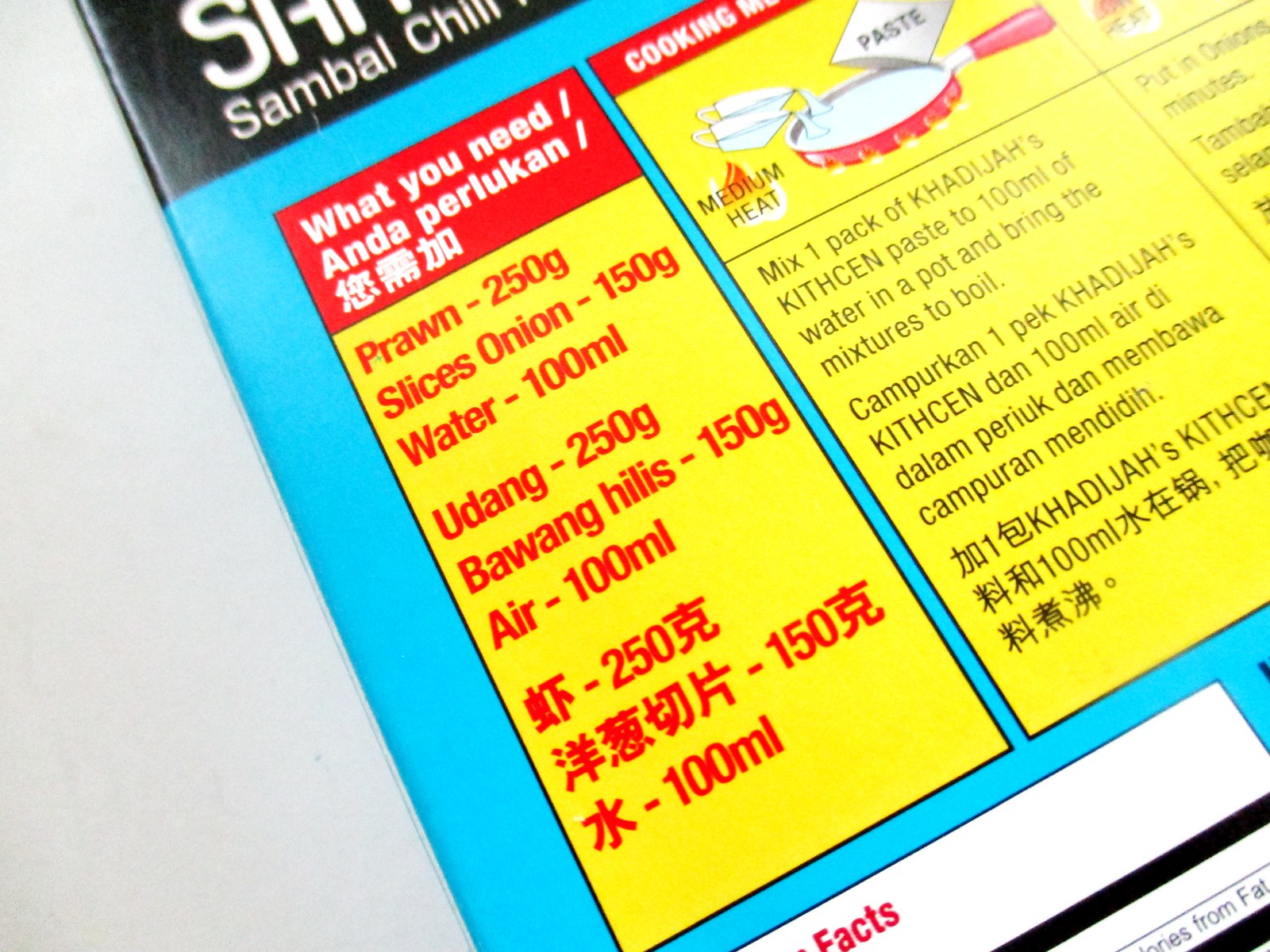The image appears to be a close-up of a recipe section, likely from the back of a food package, featuring ingredients and cooking instructions in multiple languages. Dominating the left part of the image is a vertical box with a red banner at the top stating "What You Need" and similar phrases in two other languages. Below, on a yellow background with red lettering, it lists: 

- Prawn, 250 grams
- Slices of onion, 150 grams
- Water, 100 milliliters 

These are followed by the same ingredients in two different languages. To the right, partially cut off, is a larger yellow rectangular box segmented into sections detailing the cooking instructions. The recipe instructs to mix one pack of kitchen paste with 100 milliliters of water in a pot and bring it to a boil. Additionally, the visual elements include illustrations of pouring water and paste into a pan. The text mainly uses red and yellow colors, with some black text interspersed. This section provides a comprehensive guide to preparing a dish, suitable for store-bought paste.